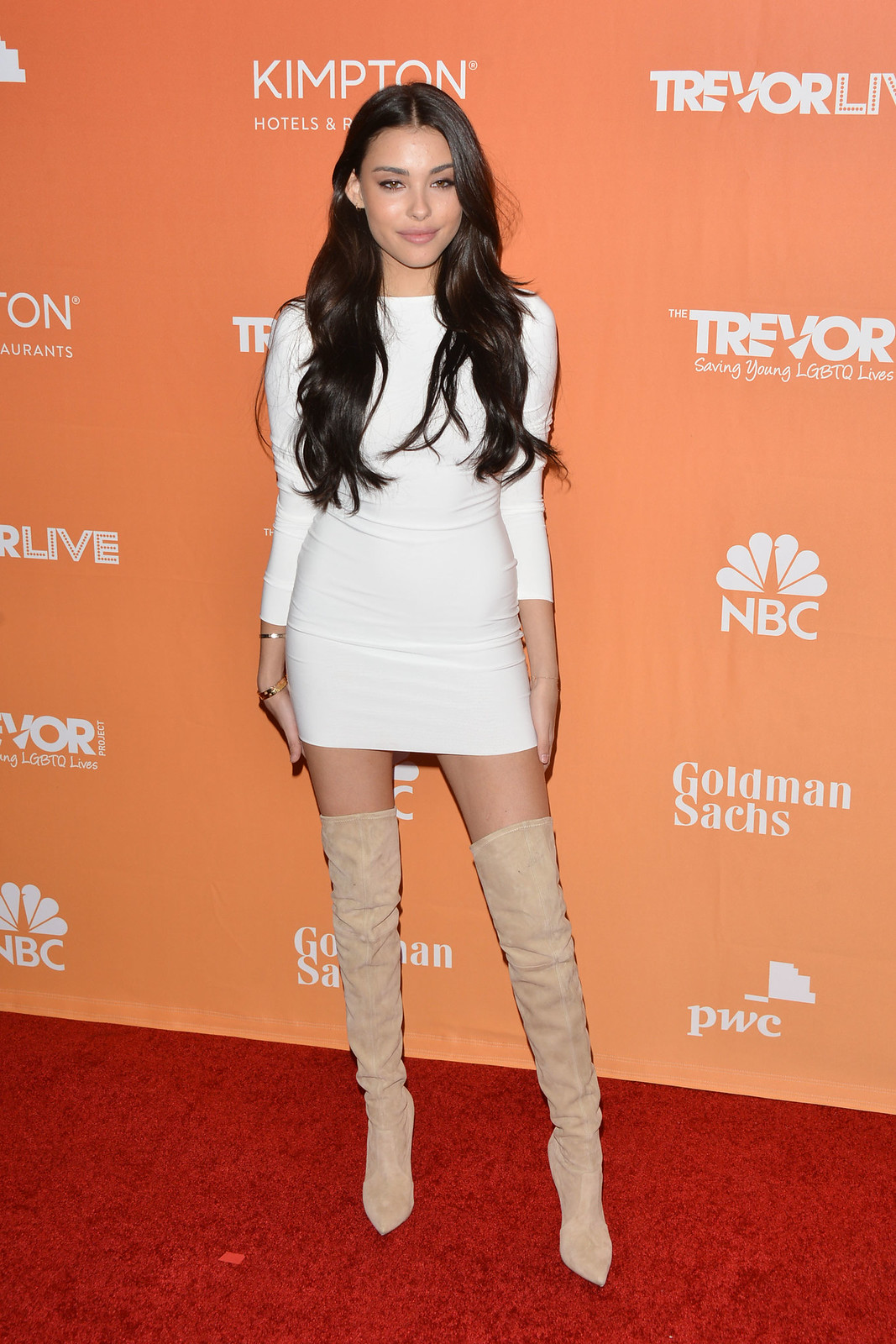In this red carpet photograph, a beautiful woman with long brunette hair cascading down past her shoulders stands gracefully against an orange backdrop adorned with numerous logos and white text. Prominent names such as NBC, complete with its iconic peacock logo, Goldman Sachs, PWC, Kimpton Hotels, and Trevor LN are visible behind her, all written in a beige hue. The floor she stands on is a vivid red, typical of celebrity events. She is dressed in an elegant, tight white mini dress with long sleeves that barely reaches her thighs. Complementing her outfit, she wears tan thigh-high leather boots with high heels, which accentuate her legs. She accessorizes her look with gold bracelets on her right hand, which she holds down by her side, gently holding her skirt. Her radiant smile completes the captivating image of a poised and stylish celebrity or model.